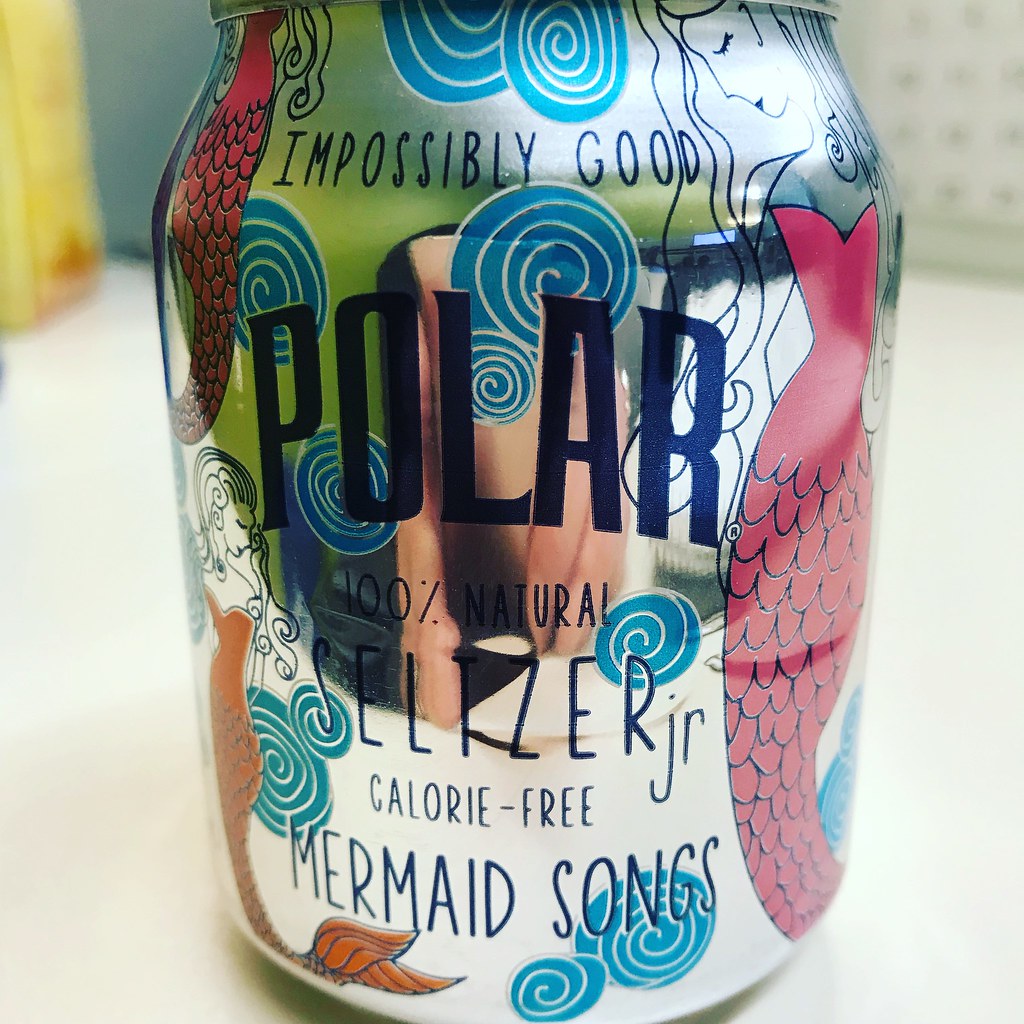This vibrant color photograph captures an 8-ounce can of Polar Seltzer, Jr. The can, made of silver aluminum, features an enchanting design adorned with mermaids. These mermaids, detailed with red tops and tails, gracefully swim around the can, adding a touch of whimsy to the packaging. Notably, one mermaid positioned near the bottom left corner sports an orange top and tail, standing out amidst the others. Complementing the mermaid motif, blue swirly shapes reminiscent of seashells accentuate the can's nautical theme. The front of the can proudly displays the brand name, Polar, along with the slogan "Impossibly Good Polar Seltzer, Jr." It also highlights key attributes of the beverage: "100% natural" and "calorie-free." The can sits elegantly on a pristine white surface, making its lively design pop even more.